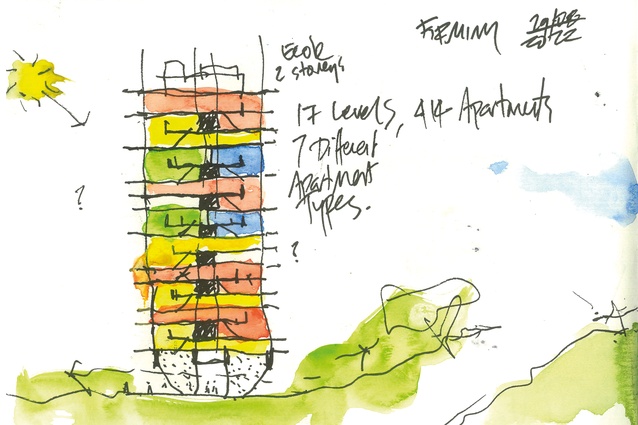The image appears to be a colorful, impressionistic watercolor painting, possibly created by a child. Dominating the scene is a tall, multi-story building characterized by vertical stripes in red, green, blue, and yellow, visually indicating different floors. Cursive handwritten text spans the painting, though somewhat illegible, referencing details such as "two-story," "17 levels," "414 apartments," and "seven apartment types." The foreground features splotchy green patches representing grass, while a yellow splotch in the top left corner likely symbolizes the sun. Additional elements include squiggly lines suggesting mountains, paths, or fields, and a small patch of blue possibly depicting the sky. Despite its chaotic and impressionistic style, the painting intriguingly attempts to convey architectural details amidst colorful, abstract elements.